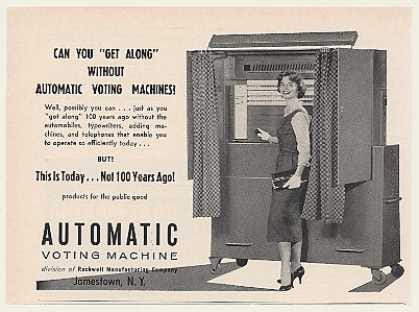This is a vintage black-and-white advertisement for an automatic voting machine, likely from the 1940s, showcasing a woman in a classic dress, high heels, and a white blouse, standing at an old-style voting machine. The background has a discolored look, mostly gray with hints of off-yellow. The smiling woman is interacting with the machine, possibly adjusting one of the dials. She holds a black clutch bag in one hand. The advertisement's text prominently asks, "CAN YOU 'GET ALONG' WITHOUT AUTOMATIC VOTING MACHINES?" in large, bold letters, followed by smaller text hinting at technological advancements by comparing it to living without automobiles and typewriters 100 years ago. It concludes with "Products for the public" and identifies the manufacturer as the Automatic Voting Machine Division of Rockwell Manufacturing Company, based in Jamestown, New York.